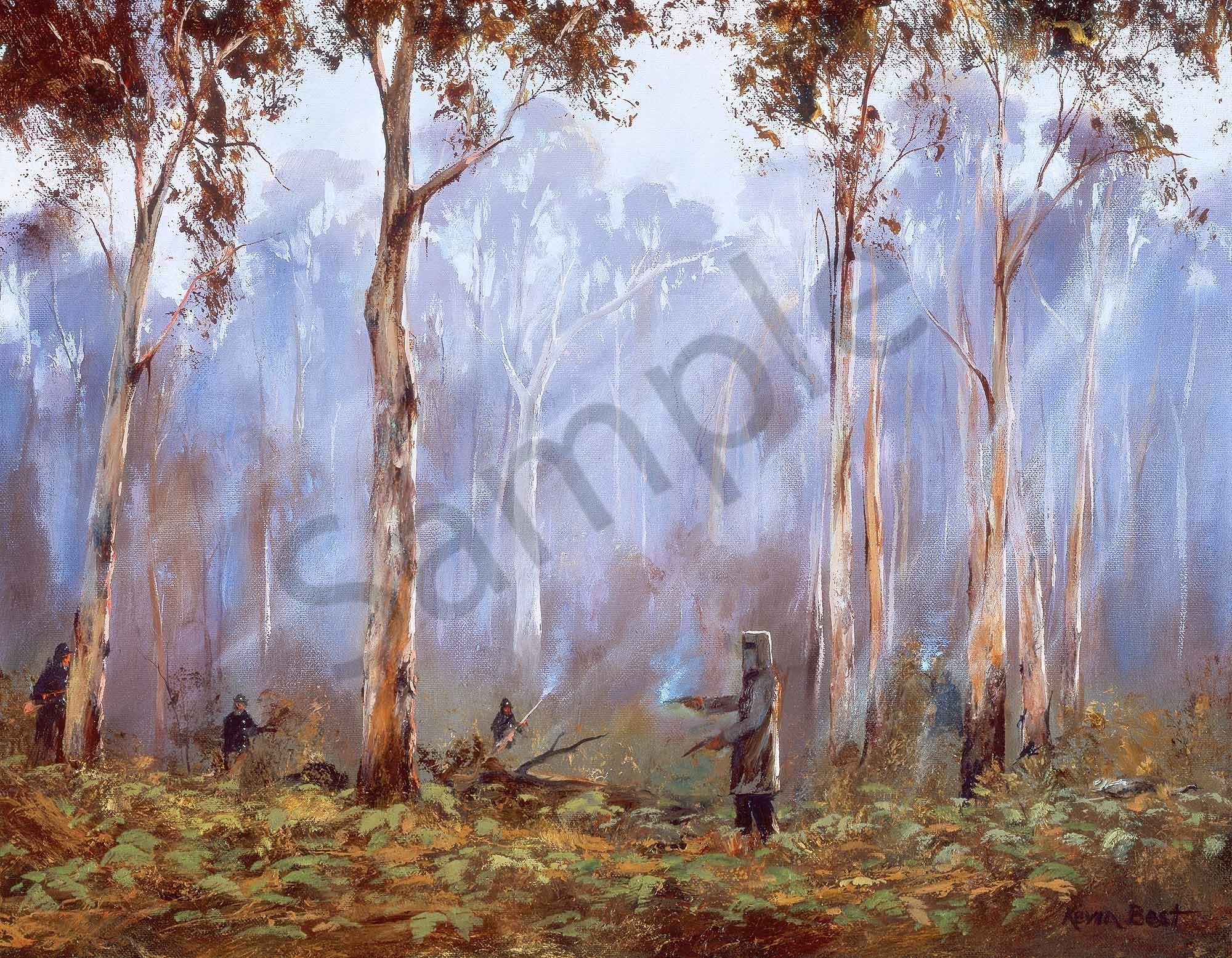This detailed painting captures an intense forest scene, steeped in historical drama. Central to the composition is a figure clad in a distinctive homemade armored suit, reminiscent of the infamous Australian outlaw, Ned Kelly. The suit includes a cylindrical helmet with a narrow slit for vision. This enigmatic character is brandishing two smoking guns, one in each hand, adding a palpable sense of immediacy and tension. Surrounding him are several figures in dark blue or black uniforms, likely representing pursuing law enforcement officers, each armed with rifles and appearing in combat-ready stances. The forest itself is densely packed with tall, mostly bare trees, their sparse foliage showing hints of brown and green. The forest floor is thickly covered in leaves, ranging in color from green to orange to brown, enhancing the autumnal feel of the scene. The background has a gray, smoky hue, suggesting recent gunfire or a tension-filled atmosphere. Diagonally across the painting, a watermark reads "sample," and the lower right corner bears the artist’s name, Kevin Best.